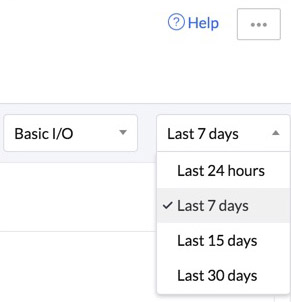The image appears to be a small snippet of a software interface, likely a dashboard or data visualization tool. The focal point is a drop-down menu located in the upper right-hand corner, dedicated to setting a specific time frame for data analysis. This menu displays several options, with "Last 7 days" currently checkmarked. Additional options within the drop-down include "Last 24 hours," "Last 15 days," and "Last 30 days." Towards the right, there's another toggle menu labeled "Basic I/O" that has not been expanded. Dominating the uppermost section of the image, there's a prominent "Help" link, represented in blue text alongside a question mark icon. The overall color scheme of the interface is predominantly white, with black text used for the majority of labels and information, except the blue colored "Help" link, adding a visual distinction.